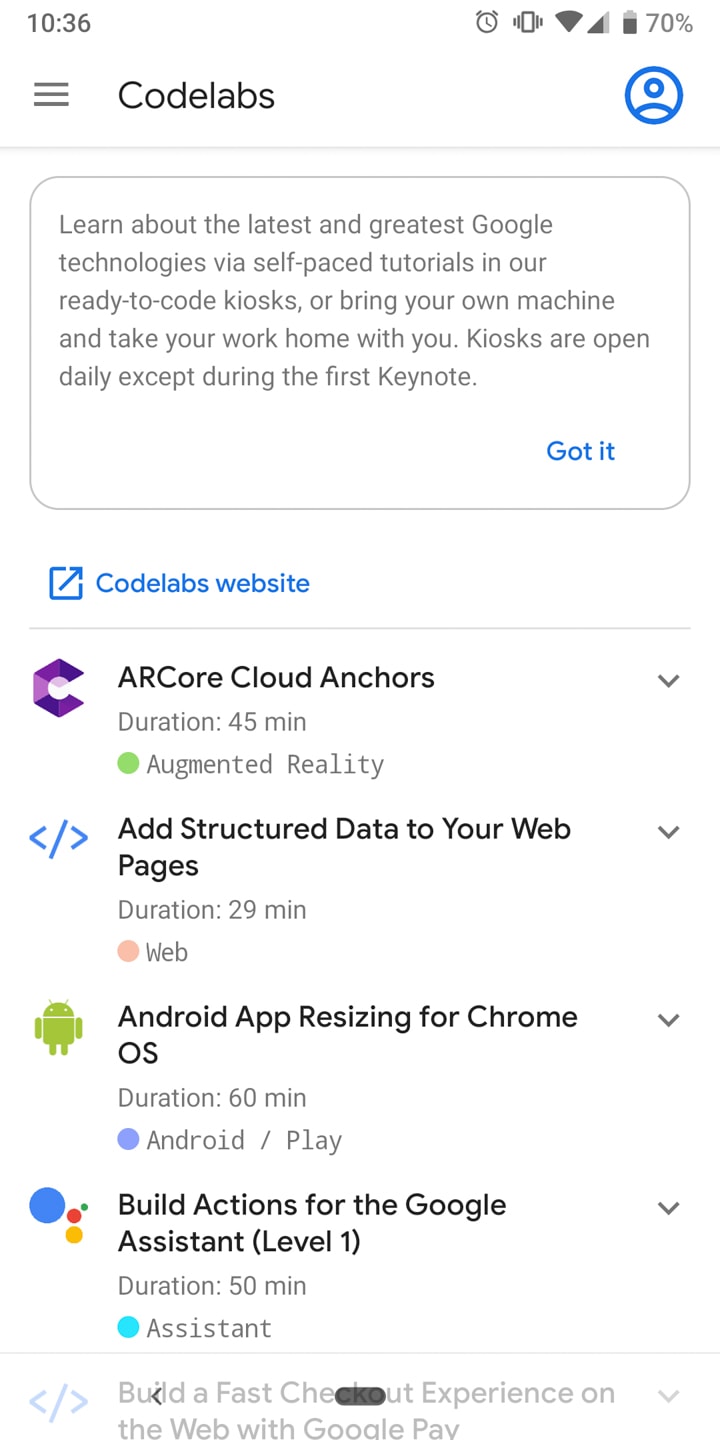The image features a clean white background. At the very top of the image, the number "1036" is displayed. On the right side, there's a phone status bar showing a 70% battery level. Below this, in black text, the word "CodeLabs" appears, followed by a blue icon depicting a person.

Centered beneath this is a gray-outlined rectangle with a white interior, maintaining the white background theme. Inside this rectangle, in gray text, it reads: "Learn about the latest and greatest Google technologies via self-paced tutorials in our ready-to-code kiosks, or bring your own machine and take your work home with you. Kiosks are open daily, except during the first keynote." In the bottom right corner of this box, there is a blue button labeled "Got It."

Beneath this rectangular box, there is blue text that reads "CodeLabs website." Following a thin underline, additional black text lists various learning modules with durations and categories:
 
- "ARCore Cloud Anchors, duration 45 minutes, augmented reality."
- "Add structured data to your web pages, duration 29 minutes, web."
- "Android app resizing for Chrome OS, duration 60 minutes, Android Play."
- "Build actions for the Google Assistant, level one, duration 50 minutes, assistant."

Finally, along the bottom edge of the image, it states: "Build a fast checkout experience on the web with Google PAV."